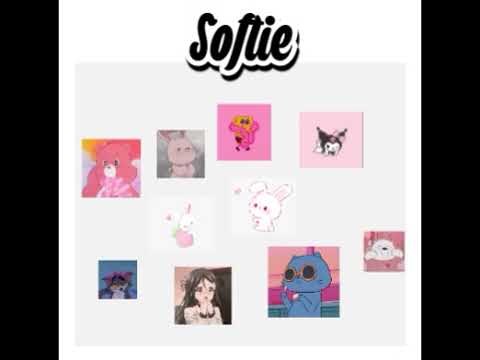The image, resembling an advertisement, is a small, horizontally rectangular graphic divided by wide black rectangles on both sides, with a clean white background in the middle. At the top, the word "Softy" is elegantly written in cursive black letters with a white outline. Below this text, the central section is populated with a series of eight small, vibrant pink squares and rectangles, each containing various cartoon characters. These squares are arranged in two rows, with three squares on the top row and two on the bottom, separated by two faint pink images of bunny-like creatures. 

In the top row, starting from the left, the first square showcases a pink Care Bear, the next one has a pink bunny, followed by an image that appears to be Spongebob. To the right of Spongebob's square is another cartoon animal in a pink robe, and finally, a pink square featuring another cartoon character. In the bottom row, starting from the left, the squares feature a dark-haired girl with her hands to her mouth, a creature that looks like a blue cat wearing orange-framed sunglasses, and another light-colored cartoon creature. The faint pink images between the rows subtly blend into the white background, further defining the whimsical and artistic nature of the piece.